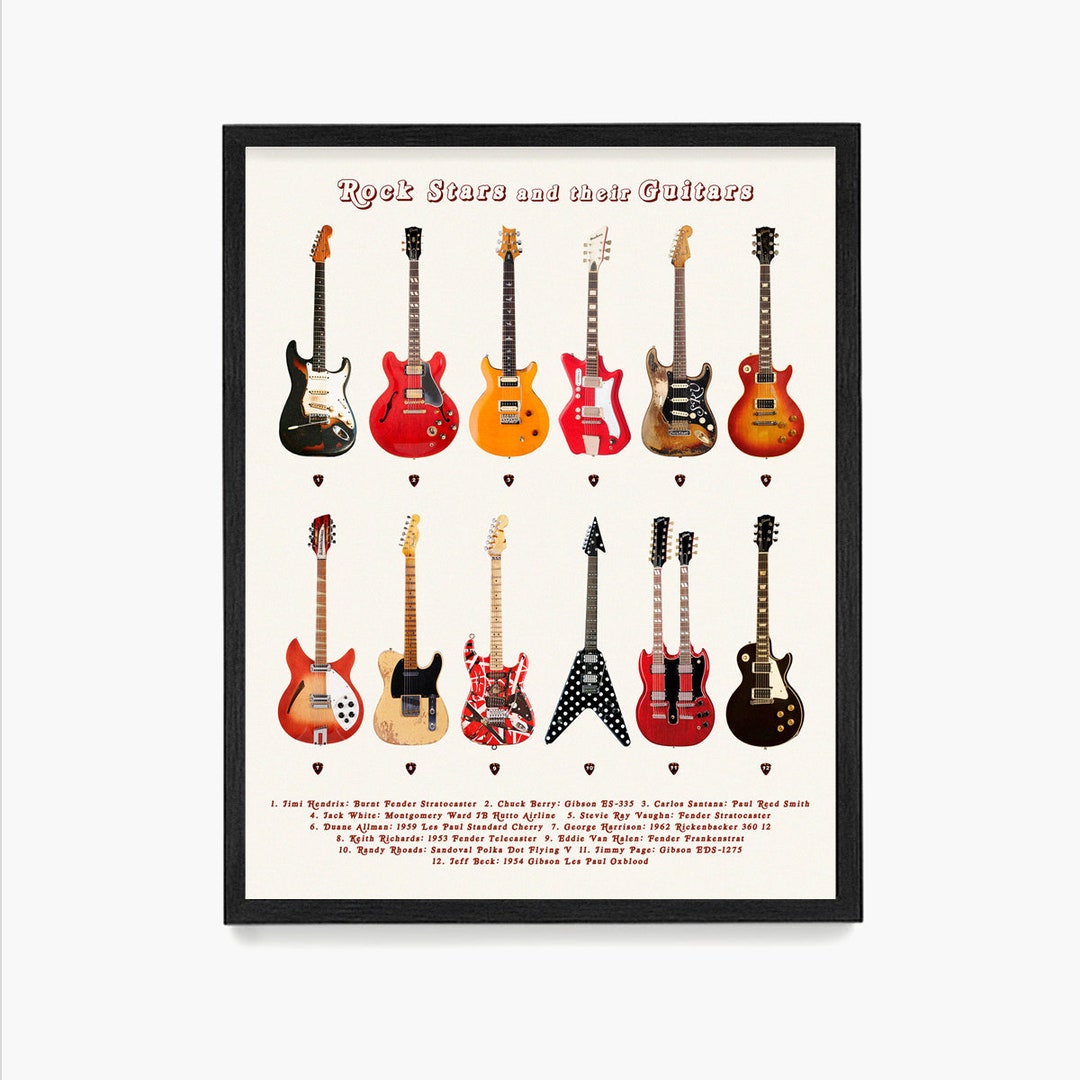This image displays a poster with a black wooden frame against a white background, showcasing a collection of twelve iconic electric guitars arranged in two rows of six. At the top, bold white text with a reddish outline reads "Rock Stars and Their Guitars." Each guitar in the image is unique, featuring a variety of colors and designs such as black, red, yellow, and even a spotted black and white pattern. Noteworthy among them are guitars belonging to legends like Jimi Hendrix, Chuck Berry, Carlos Santana, and Jack White. Some of the guitars include distinctive styles, such as a double-necked red guitar and a square-shaped guitar. Below each guitar, small guitar picks are visible, and at the bottom of the poster, red text attempts to identify the guitars, although the text is too small to be easily read.